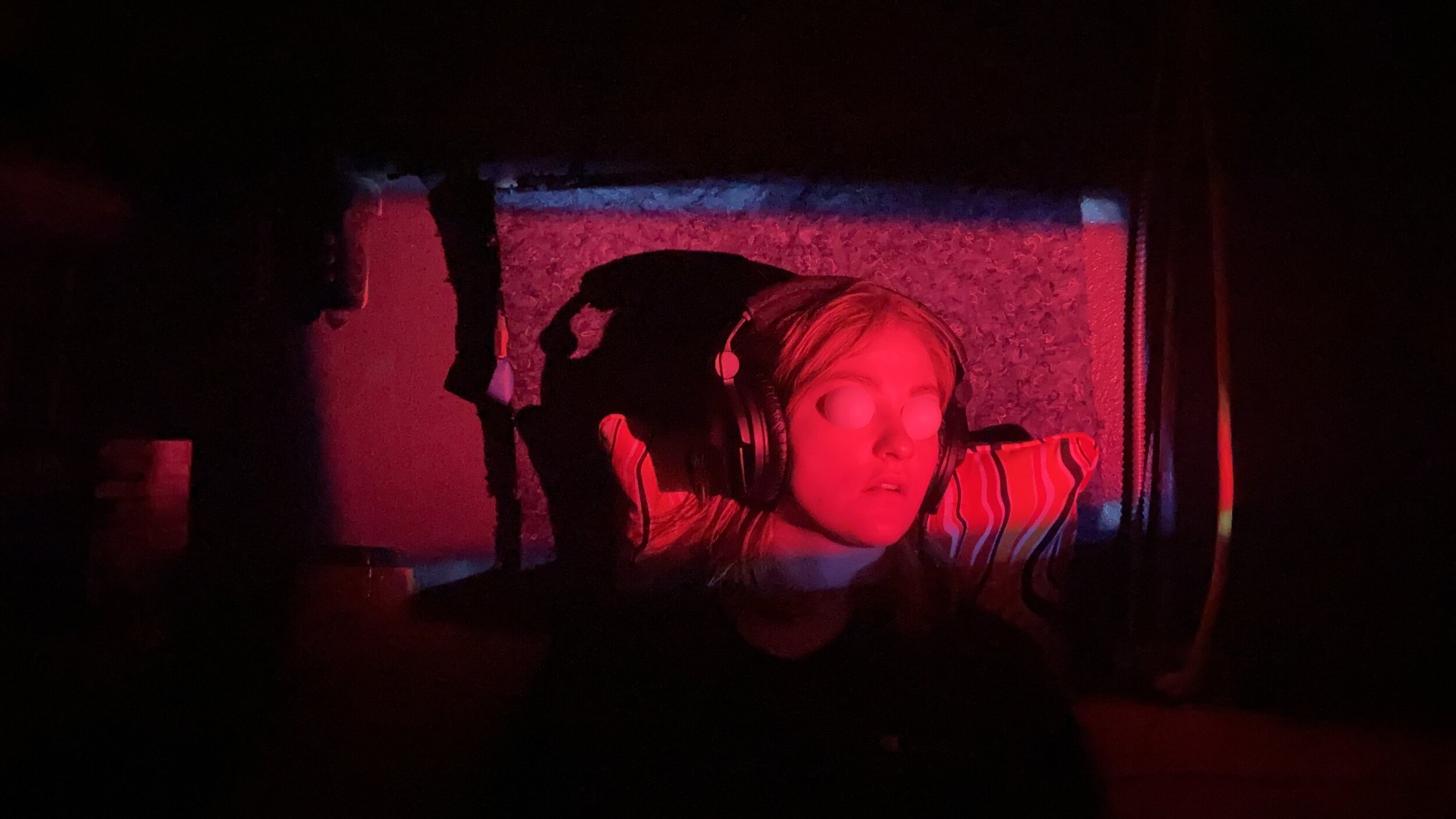The image depicts a woman with long blonde hair, seated in what appears to be a dark room. She is wearing large, black headphones and has a striped pillow behind her, suggesting she might be in a seat or bed. Her eyes are covered with objects resembling eggs or eye gels, giving her a peculiar appearance. A bright red light highlights her face, creating a stark contrast against the surrounding darkness. The woman has a shocked or distracted expression and appears to be leaning slightly, possibly against a headboard. The focus of the image is centered on her illuminated face, making the rest of the background obscure and indistinguishable.